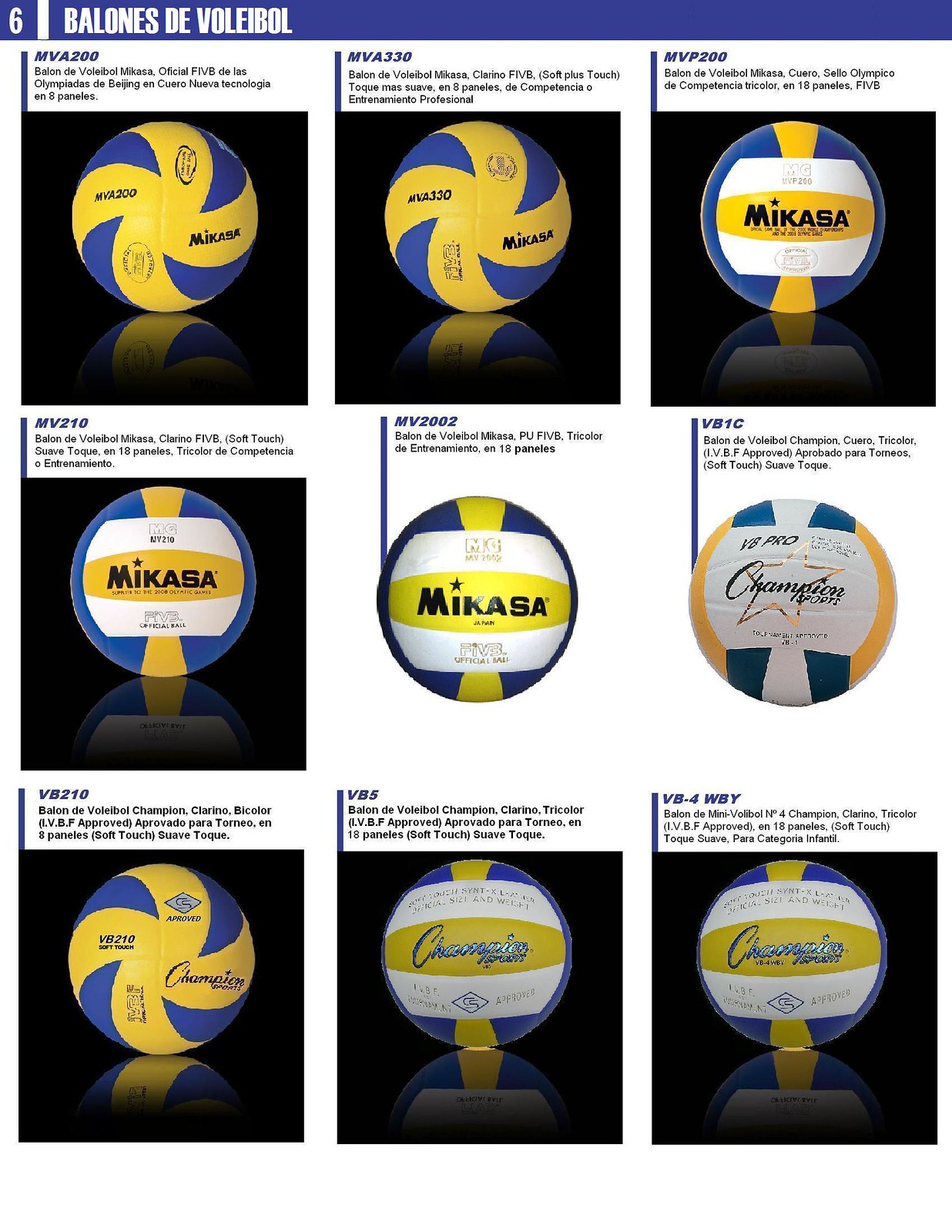The image showcases a product page for various volleyballs, arranged in a 3x3 grid with nine smaller images. At the top of the page, there is a blue bar spanning the entire width, featuring the white text "Balones de Volei" along with the number six in a small blue square on the left. Each volleyball image is accompanied by its name and a brief description. 

The volleyballs present a mix of blue, yellow, white, and sometimes orange color combinations, designed with stripes, swirls, and large central panels. The first row features volleyballs predominantly in blue and yellow with black backgrounds, except the third ball which has a white background with the brand name "MIKASA" in black text. The second row includes similar designs; the first ball mirrors the third ball from the top row with a black background, followed by another "MIKASA" ball but with a brighter yellow and a white background. The last ball in this row has a unique combination of white, blue, and orange with an unspecified logo. 

The bottom row mirrors the top's arrangement: the first ball is similar to the top left, the second ball has a white background with blue and yellow stripes and the word "champion" written in blue cursive, and the last ball on the bottom row is identical to it.

Most backgrounds are black except for three: the center and right images in the middle row, and the second ball from the left on the bottom row. The various volleyball designs feature prominent branding and color patterns that cater to different preferences and styles.